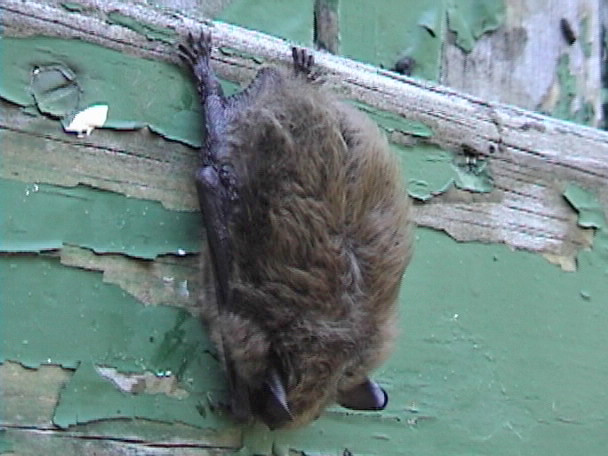This full-color, square photograph captures a close-up nature scene taken outdoors in daylight. The central focus is a small, medium-brown bat hanging upside down from an old, peeling green-painted wooden wall. The bat's back is prominently featured, with its black ears and tiny dark brown legs visible, while its wings remain folded. The green paint on the wall is significantly chipped, revealing the age and wear of the wooden surface. In the upper left corner of the image, a large screw can be seen embedded in the wood. The bat clings to the wall with its hands, displaying its small fingers as it hangs from the side of the structure.